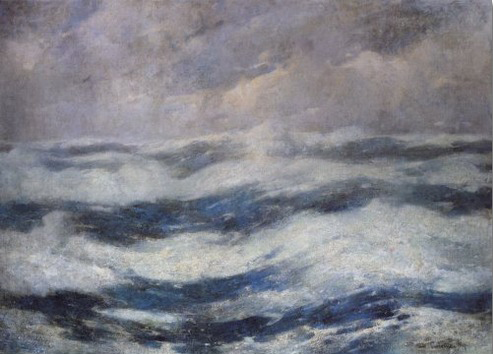The painting portrays a tumultuous ocean scene, capturing the raw power and chaos of a stormy day at sea. The majority of the image is dominated by the vividly textured water, which is characterized by an intricate pattern of aggressive, zigzagging waves. The waves, with their white crests, seem to be charging towards the observer, displaying a dynamic mixture of dark gray and blue hues. The water is more white than blue, emphasizing the intensity of the sea's turmoil, likely stirred up by powerful winds. 

In the background, the sky is painted with swirling clouds that are dark gray and ominous, occasionally interrupted by flashes of light that suggest lightning. The clouds appear wild and wind-driven, enhancing the overall feeling of a fierce storm. Despite the storm's ferocity, about 40% of the composition is dedicated to the sky, allowing for a sense of depth and distance as the storm recedes into the horizon. 

To the right bottom corner of the painting, a small rock emerges from the churning waters, adding a touch of detail and grounding the scene in a bit of reality. The artwork, although highly realistic and detailed, retains an unmistakable artistic touch that distinguishes it as a painting rather than a photograph, capturing both the beauty and terror of a stormy sea.